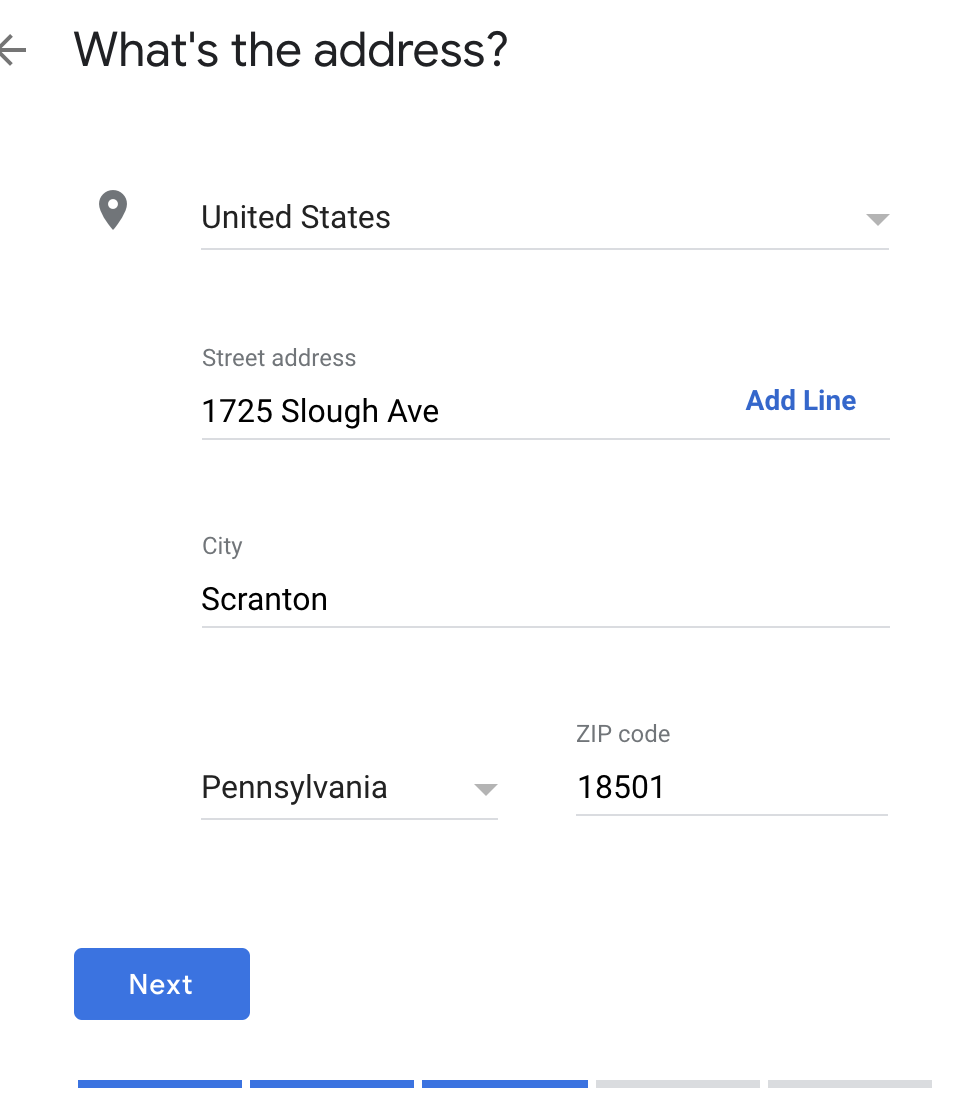A screenshot, likely from a mobile device, captures a user interface for entering an address. At the top, there's a back arrow icon followed by the text "What's the address" in black. Below, a grey location icon precedes a text box with "United States." The text box features a grey drop-down arrow. Further down, there's a field labeled "Street Address" with "1725 Slough Ave" written in grey. Next to it, a blue headline text appears. Below that, the city field is marked "Scranton" in black within a grey-bordered text box. The state, "Pennsylvania," is in black with a drop-down arrow beside it. Lastly, the ZIP code field shows "18501," followed by a "Next" button in white text on a blue background.